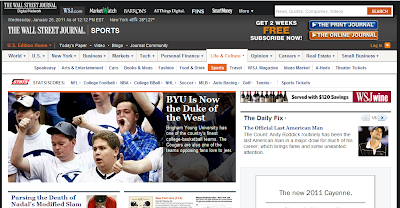The screenshot is a cropped, low-resolution capture of what seems to be the Wall Street Journal's sports section. Due to the extreme zoom-out, details are minimal, but it is evident that the main headline proclaims Brigham Young University (BYU) as the "Duke of the West." The comparison drawn by the article suggests that BYU has attained a level of athletic success and reputation comparable to that of Duke University, an institution renowned for its high-performing sports teams on the East Coast in Durham, North Carolina. This headline likely celebrates a significant achievement by the BYU athletic program, perhaps a championship or notable event, affirming the team's rise to prominence in collegiate sports.